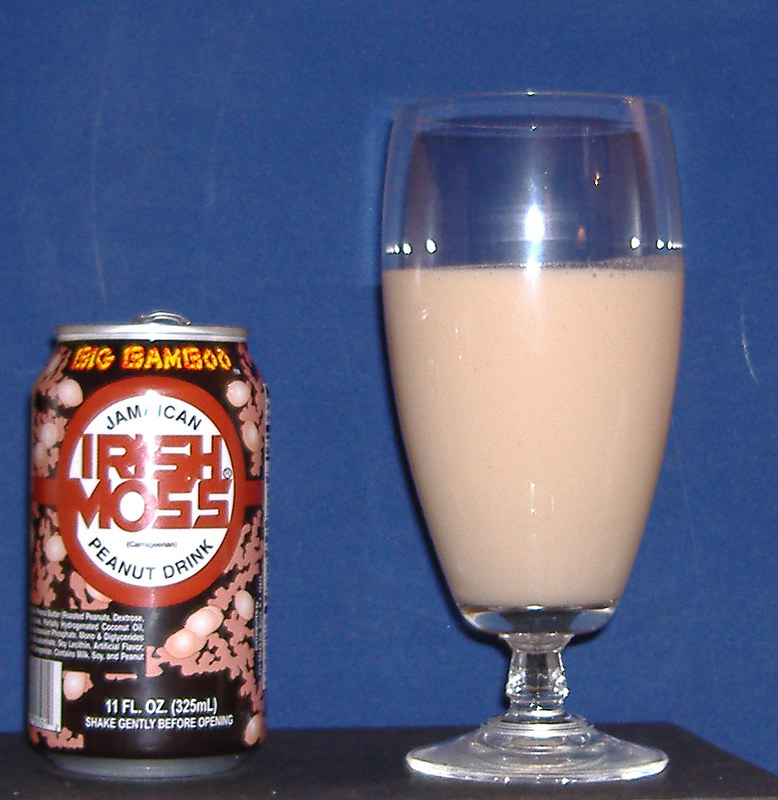This image showcases a beverage with a rich background and detailed display. The backdrop consists of dark blue wallpaper which contrasts nicely with the dark wooden platform or desk that supports two items. On the left side, there is an open can of Big Bamboo Jamaican Irish Moss Peanut Drink. The can features a predominantly dark brown color with light pink and pinkish-red designs scattered across it. A notable red circle frame surrounds the inner white label, where the product's name is printed. The words "Jamaican" and "Peanut Drink" appear in smaller black print, while "Irish Moss" is highlighted in larger, red print. Additional information about the drink's flavors, ingredients, and a barcode can be found lower down on the can. It also states "11 fluid ounces (325 milliliters)" and "Shake gently before serving" in white lettering. To the right of the can, a tall, clear white glass stands, filled more than halfway with what appears to be the peanut drink. The beverage has a beige-ish pink hue, adding to the image's overall aesthetic appeal.